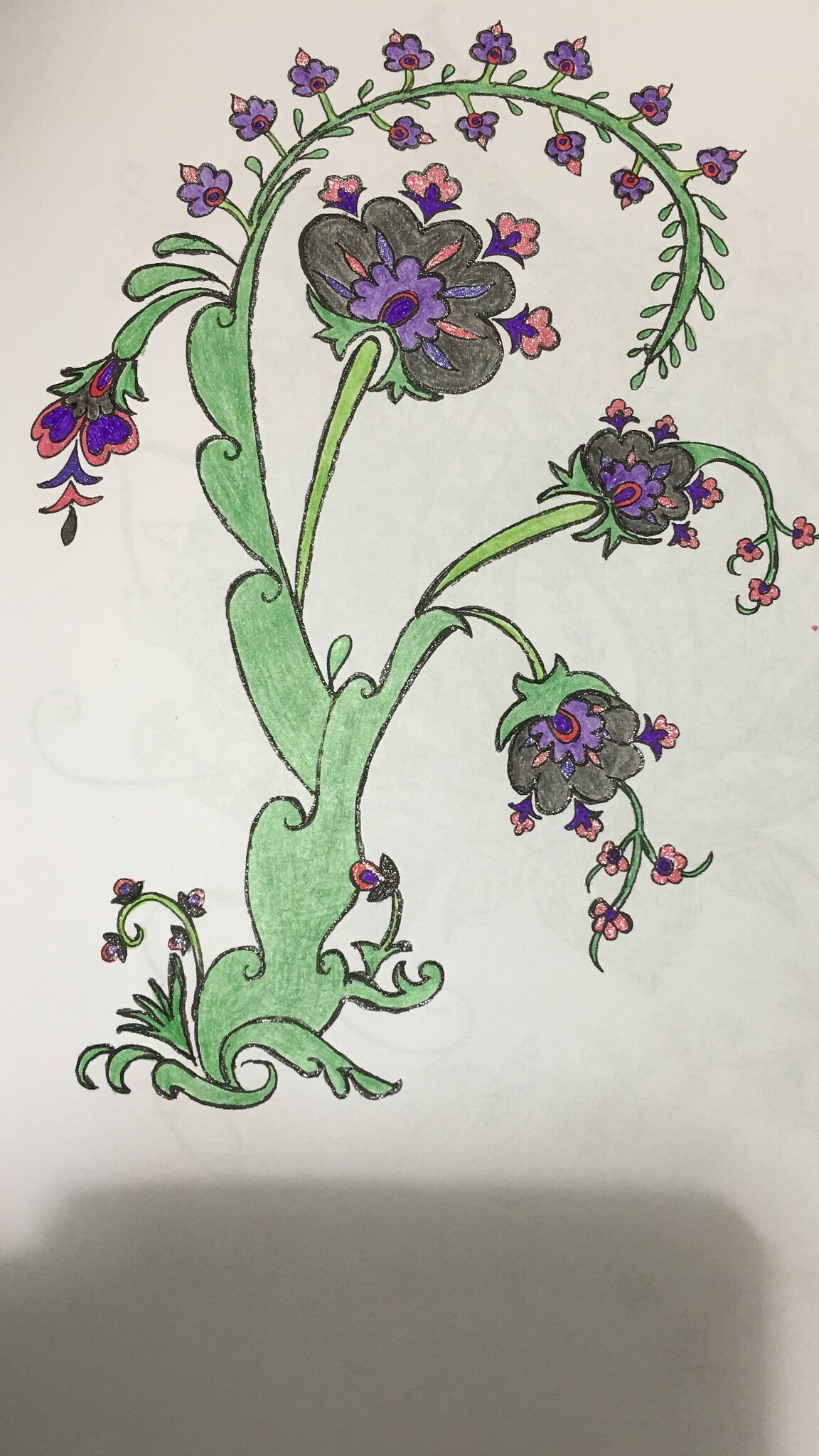This image is a real-life photograph of a drawing rendered on white paper. The centerpiece is a peculiar plant characterized by wavy and wobbly stems, drawn with a distinct black outline. The artist used an array of crayons or colored pencils to bring the plant to life, showcasing various smaller buds and flowers at the ends of the numerous stems. Some flowers are small and feature purple petals with red centers, while others display a dark greenish-gray hue with purple interiors and pink accents. Scattered among these are little pink flowers adorned with dark purple spots. The entire drawing captures a whimsical and colorful botanical scene. A prominent rectangular shadow, likely cast by the photographer's phone due to overhead lighting, is visible at the bottom of the image, adding an unintended dimension to the composition.